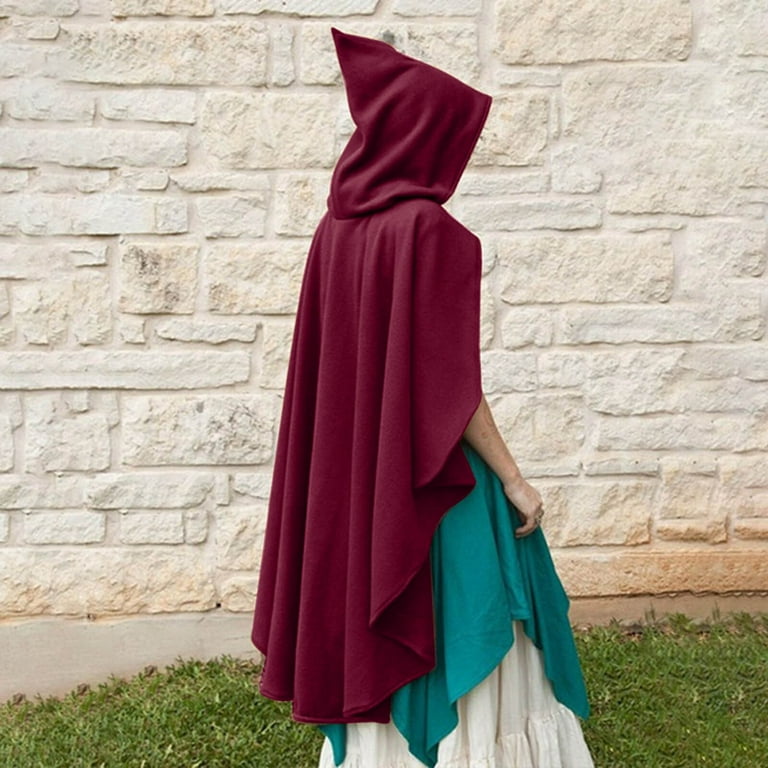A mysterious figure stands against an irregular, whitewashed stone wall, with vibrant green grass at the ground. The person, possibly a young woman, wears an elaborate outfit consisting of a maroon-colored, pointed hooded cape that drapes down to their knees. Beneath the cape is a deep turquoise dress, and beneath that, a white, pleated, and fringed dress that reaches down to their ankles. Only the right arm is visible, extended slightly with a large ring on the ring finger. The person's face is completely obscured by the hood, adding to the enigmatic and possibly magical or witch-like aura of the scene. The setting's details—the texture of the stones, the green of the grass, the pale skin of the figure—add to the captivating and somewhat eerie atmosphere.